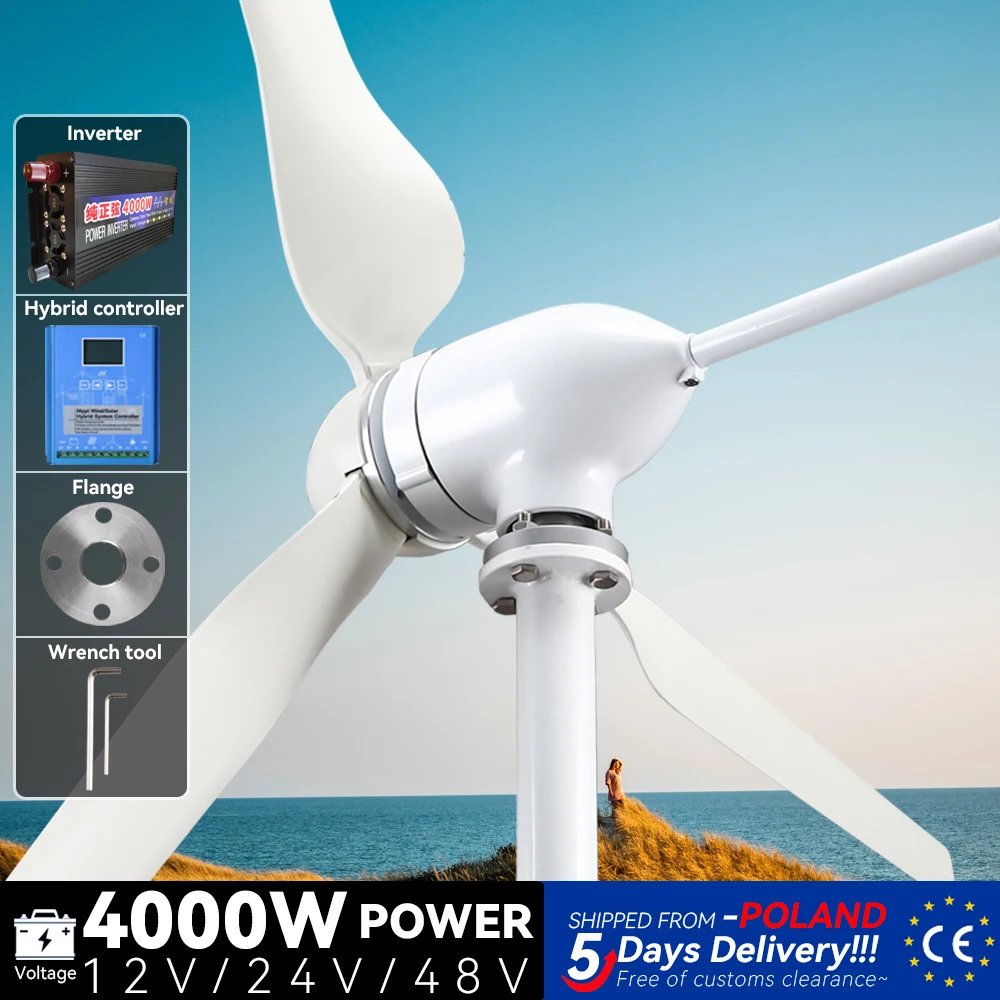The image is an advertisement for a wind turbine, prominently featuring various components and key specifications. The scene is against the backdrop of a serene beach with dried-up grass and a woman standing on a beige grassy hill, gazing over a calm blue ocean under a light blue sky with hazy white clouds. The wind turbine, resembling a white windmill, faces slightly away from the camera towards the left.

Overlaying the image are four gray stacked boxes on the left-hand side, each containing text and a relevant picture. The top box is labeled "Inverter" and displays a black box. The second box says "Hybrid Controller" with an image of a blue circuit board. Below that, the third box mentions "Flange," showing a silver circular piece with holes. The last box displays two silver Allen wrenches under the label "Wrench Tool." At the image's bottom, a black bar on the left notes "4000 watt power, 12 volts, 24 volts, 48 volts," and a blue bar on the right states "Shipped from Poland, five days delivery, free of customs clearance."